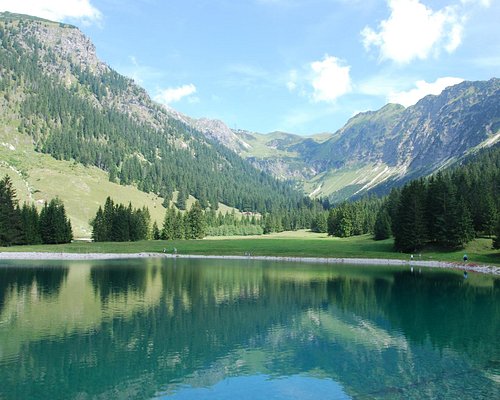The photograph captures a serene lake framed by a majestic mountainous landscape. The foreground features the tranquil water, which mirrors the towering mountains and lush greenery. On the horizon, the mountains rise prominently with rocky peaks on the right, showing a hint of snow and surrounded by sparse trees, while the left side is adorned with dense pine forests. The rocky mountain edges are bordered by a line of rocks along the lake's edge, creating a rugged outline. A narrow pathway snakes up one of the hills, adding a touch of mystery. The sky overhead is a bright blue, speckled with puffy white clouds, and a thin layer of volumetric fog lends a mystical blue mist to the distant peaks. Sunlight from the top right casts shadows and illuminates the trees and mountains, enhancing the natural splendor. The entire scene evokes a morning atmosphere, tranquil and subtly illuminated.